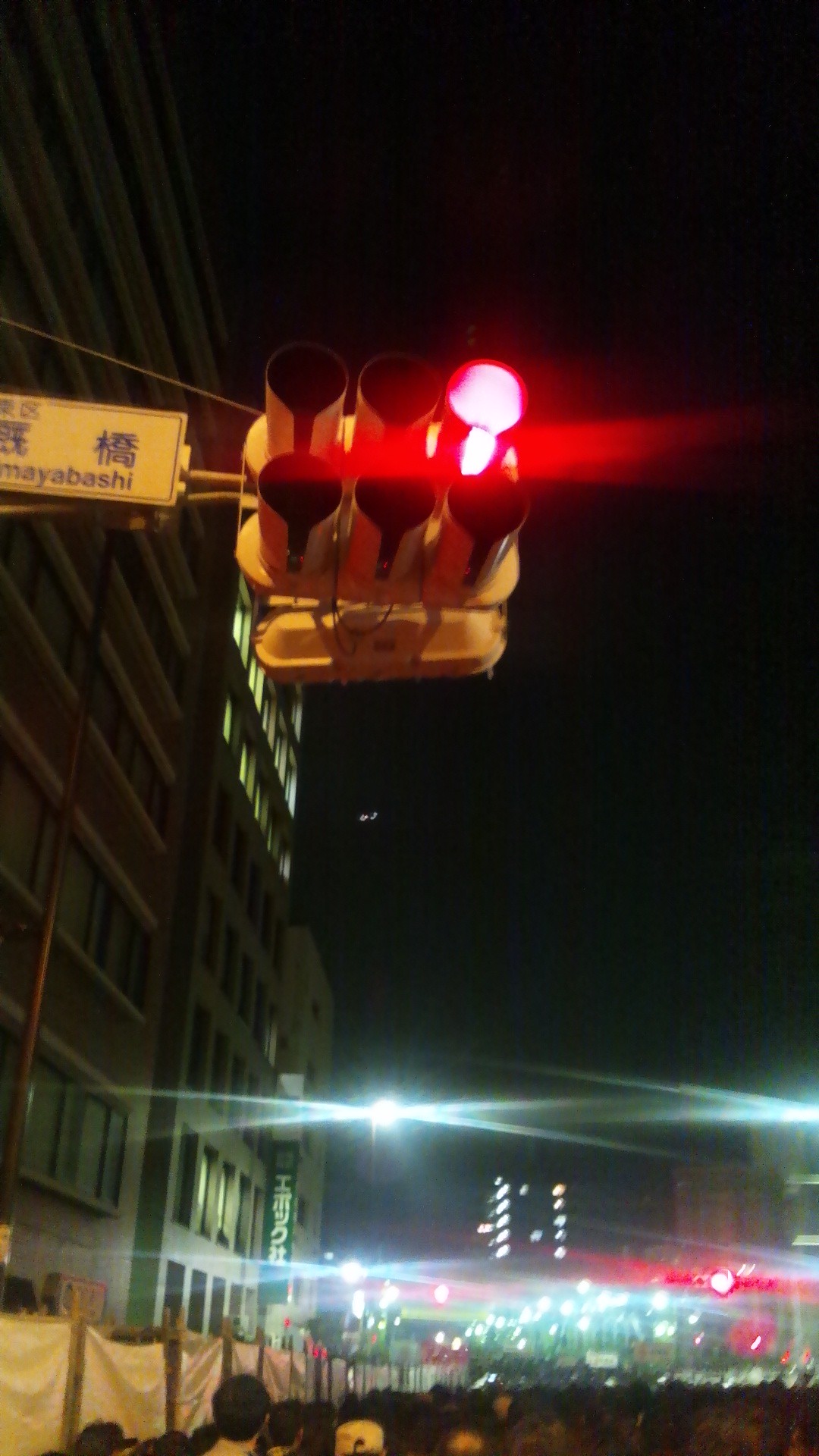The image captures a night scene in a bustling city, possibly in Japan, as evidenced by the kanji characters on a partially visible sign that hints at the name "Mayabashi." Dominating the scene is a unique stoplight featuring six circular lights, arranged in two rows of three, with only the top-right light glowing a vivid red, casting a reflective glow in the surroundings. Below this stoplight, a large crowd fills the street, with only the tops of their heads visible. On the left side of the image, tall buildings stretch up, some windows emitting light, while a makeshift white fence made of tarps supported by dark poles runs along the street. Amidst the dark sky, bright street lamps and lens flares add to the scene's urban vibrancy.